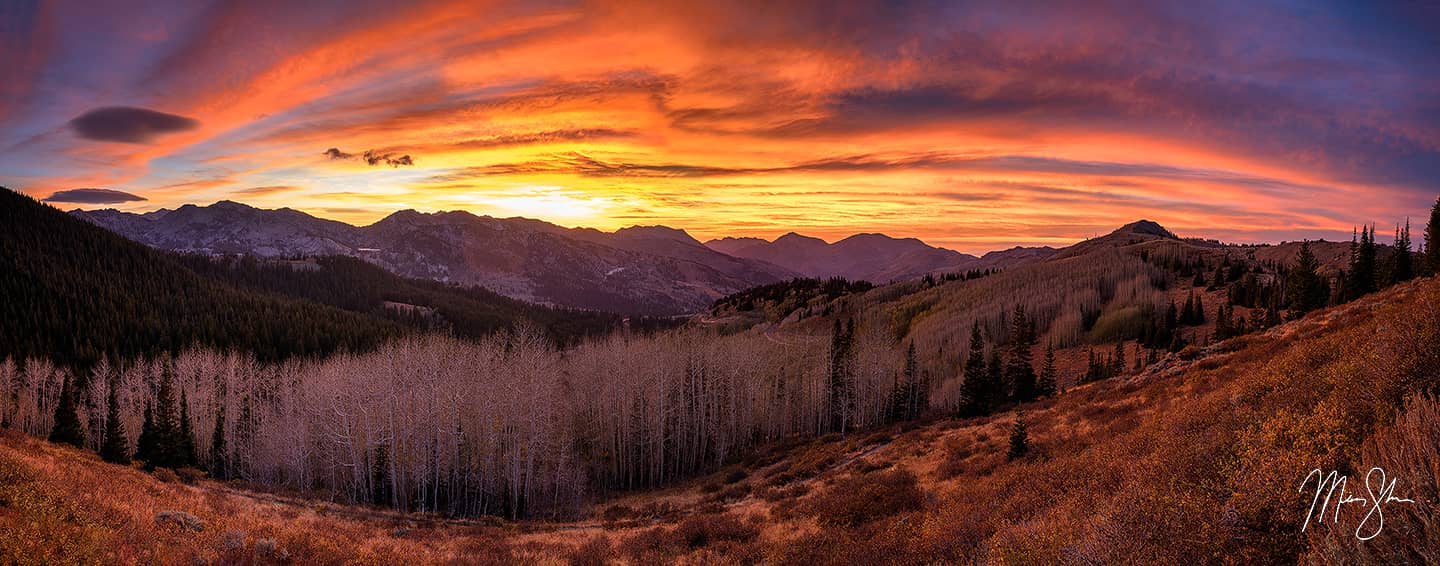This landscape painting, captured in a wide panoramic style, presents a captivating sunset scene. The sky transitions from vivid pinks and oranges along the edge of the clouds to darker shades, creating a striking contrast. In the foreground, a dusty hillside adorned with scattered green bushes and shrubs slopes down and up again, leading to a row of small trees. Beyond this, more hills covered with grass and small trees stretch towards a vast mountain range in the background, shrouded mostly in shadow. On the bottom right-hand corner of the painting, the artist's signature is visible in white. The entire scene is bathed in the warm and colorful hues of the sunset, making an engaging visual spectacle.